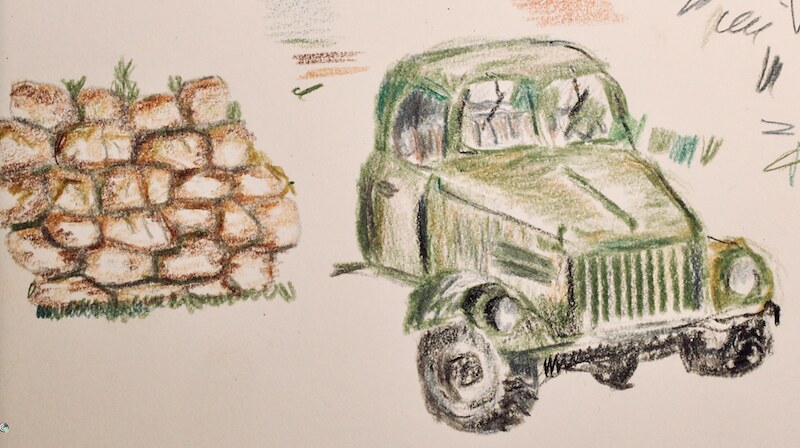This crayon drawing, created on either light tan or white paper, features a meticulously detailed scene split into two distinct halves. On the left, the artist rendered an old, weathered stone wall comprised of variously shaped rocks—circular, square, and triangular—all shaded in brown hues to add a natural, earthy feel. Between these stones, small green plants and patches of grass sprout, adding a touch of life to the ancient structure. On the right side, the focus shifts to the front of a classic vehicle that appears to be a 1950s-style pickup truck, although it bears some resemblance to a beetle or even an enclosed tractor due to its unique design. This green truck is depicted with black wheels and an axle, with the cabine and front grill drawn in metal-like detail. You can see through the clear windows to the black seats inside. Surrounding the truck, the background is scattered with colorful crayon lines and scribbles, indicating an unfinished piece but highlighting the artist's experimentation with different colors.